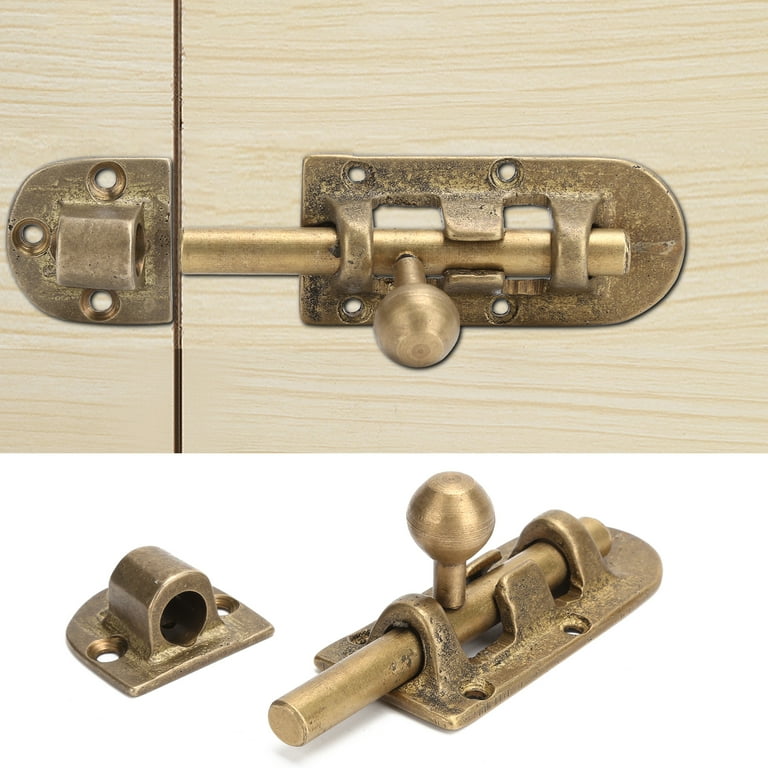This color indoor photograph features a pair of images of a vintage sliding deadbolt latch made from brass. The top image presents a top-down view of the deadbolt affixed to a light brown, maple wood surface, with visible wood grain. The deadbolt’s extended bolt portion is on the right, while the latch is on the left, though the bolt is not engaged with the latch. Below, a three-quarter view displays both pieces— the deadbolt on the right and the catch on the left. The deadbolt is a small, intricately crafted device typically suited for smaller applications like a jewelry box or a small gate. It features a knob on the slide, enabling manual operation. The bolt, or ram portion, is brass, while the holder appears to be a rough cast bronze. The locking mechanism secures by sliding the bolt into a hole on the receiving end, ensuring closure. The deadbolt has four screw mounting holes, and the catch has three, facilitating secure attachment to any wooden surface. The photographs provide detailed perspectives, showcasing both its functional positioning and isolated view for size comparison and usage understanding.